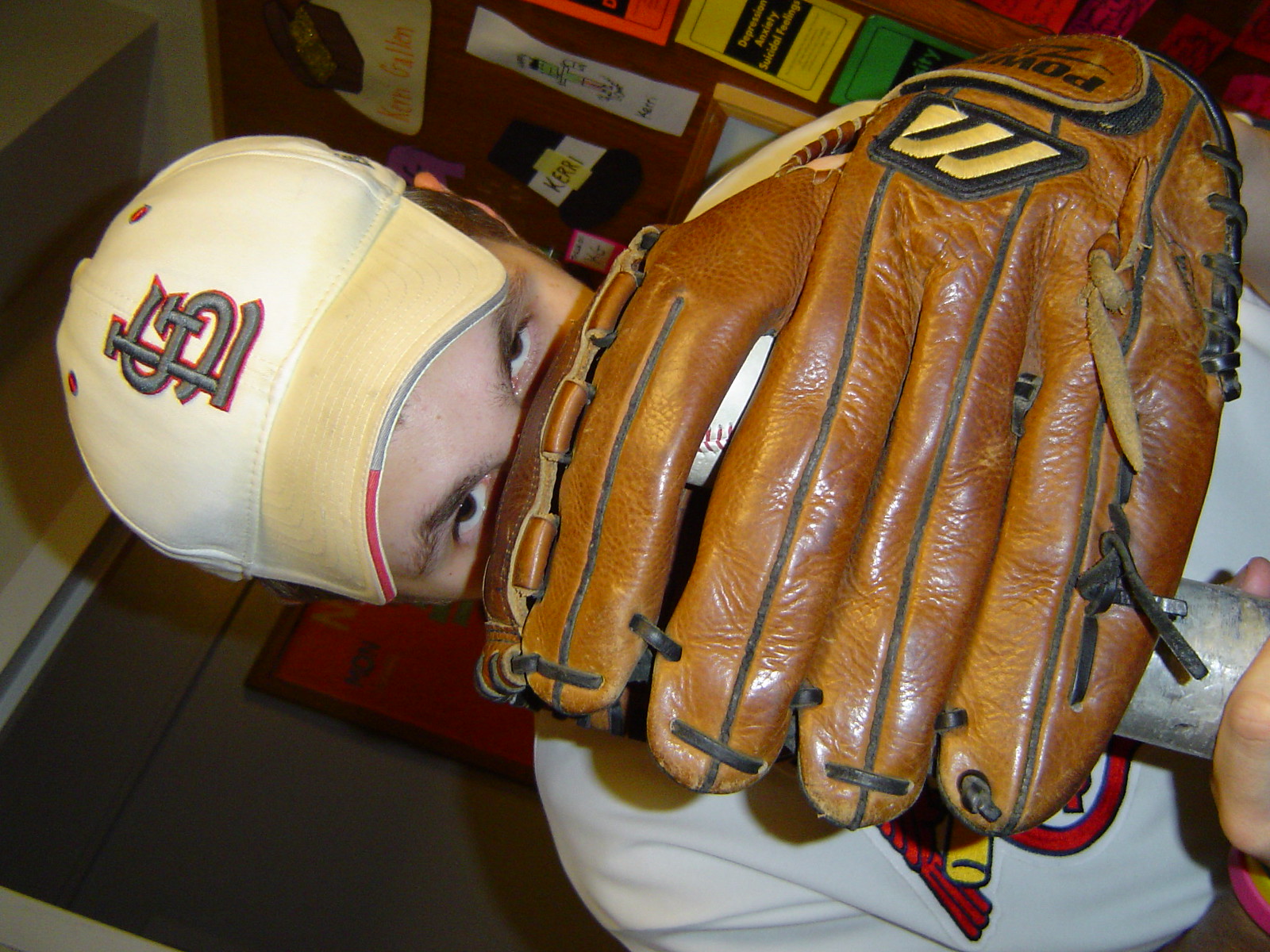The rotated photograph showcases a young man positioned sideways with a well-worn medium brown baseball glove with black laces, perfectly covering the lower portion of his face. His intense eyes peek out just above the first finger of the mitt, enhancing the eerie atmosphere of the scene. The image is rotated 90 degrees counterclockwise, transforming what would typically be a vertical portrait into a horizontal landscape. He dons a white St. Louis Cardinals baseball cap, sporting the iconic SL logo in silver with a red outline, alongside a matching jersey displaying red and yellow accents. The glove conceals a white baseball with visible red stitching between its first two fingers. The background subtly features a red door and green-yellow paper, suggesting he might be in a school setting.